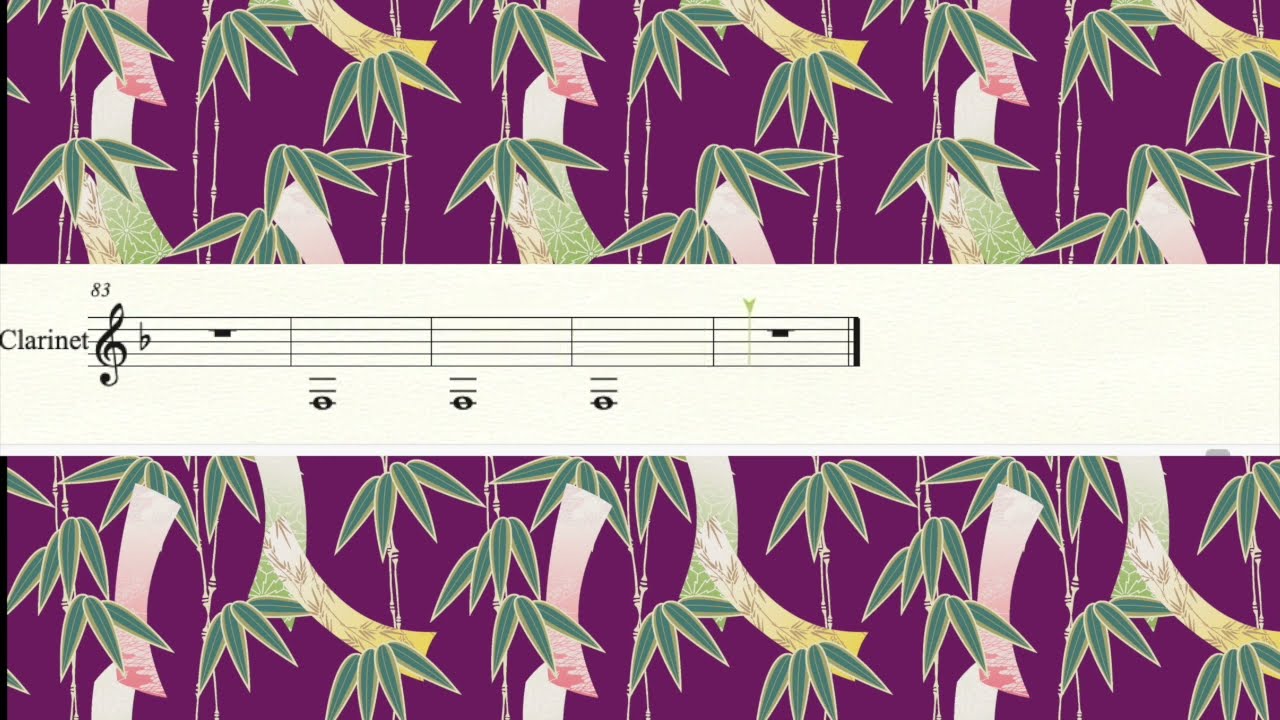The image features a digital design with an artistic, music-based theme. Centered in the composition is an off-white band containing a short piece of sheet music labeled "clarinet" on the left. The music includes traditional musical symbols, featuring a rest, three whole notes, and another rest. The background displays a repeating wallpaper pattern with a purplish-red hue, depicting stylized tree branches and leaves in green, white, and pink. This pattern spans both the upper and lower sections of the image, providing a harmonious and visually appealing contrast to the central strip of sheet music. The overall design integrates various colors such as purple, green, pink, yellow, black, and white, contributing to a vibrant yet cohesive artistic expression.